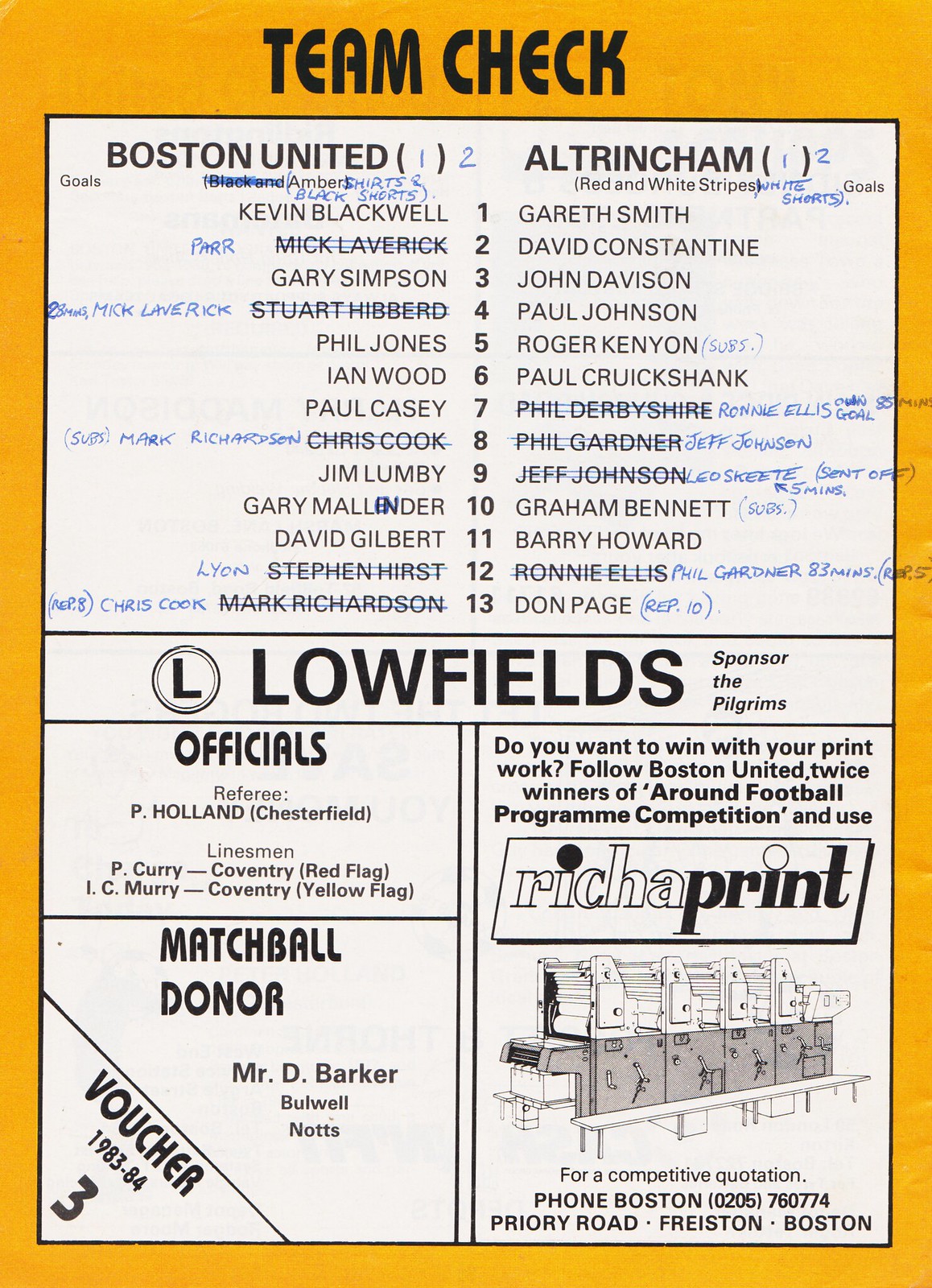The image depicts a detailed team check flyer with an orange background and a white rectangular area in the middle. At the top, bold black text reads "Team Check," followed by listings for two opposing teams: Boston United on the left and Altrincham on the right. Each side includes a list of 13 players' names and numbers, some of which are crossed out with thin blue lines and replaced with handwritten annotations, indicating player changes or replacements. Below the team listings, large capitalized text announces "Lowfields sponsor the Pilgrims." This section is followed by a list of officials and their names. Further down, the flyer identifies the matchball donor as Mr. D. Barker. The bottom left corner features "Voucher 1983-84" and the number three, while the right side contains an advertisement with the slogan "Rich a Print" and an image of a large industrial printer, promoting a printing competition that ties in with Boston United’s program.